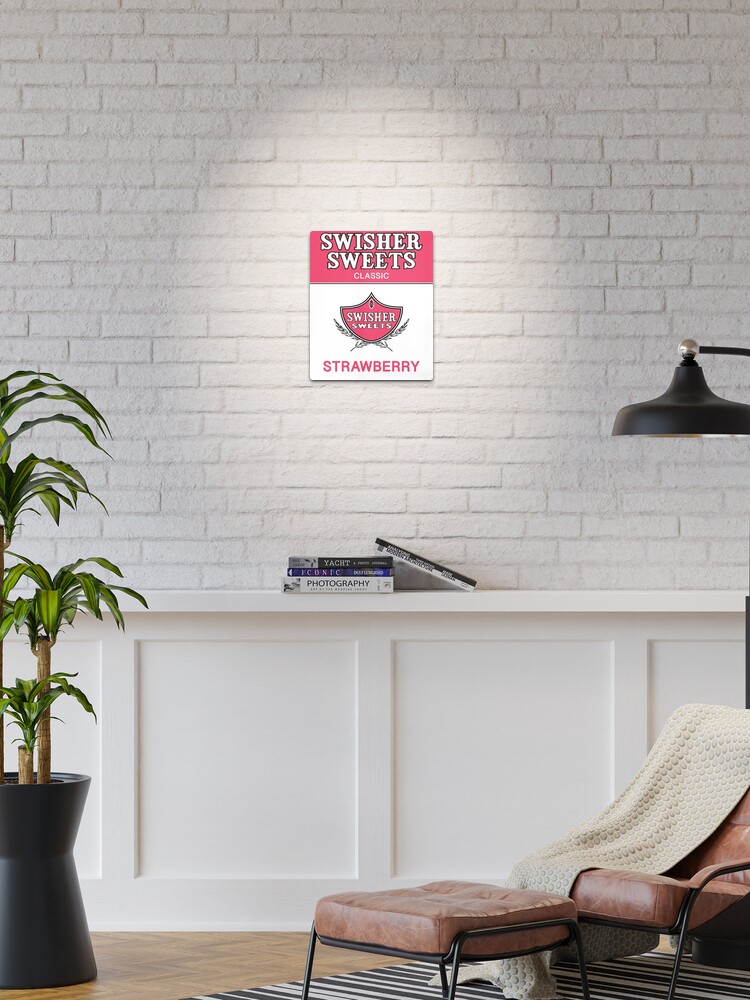The image portrays a cozy living room setting with a focal back wall that is painted entirely white, comprised of brick on the top two-thirds and wood paneling with trim on the bottom. A prominent Swisher Sweets sign hangs at the center of the brick wall. This vintage advertisement sign is divided into sections, with the top third in red, featuring the Swisher Sweets logo and the word "Strawberry" in white. The remaining two-thirds of the sign is white with red lettering. The sign is illuminated by a spotlight, making it a central element of the room's decor.

Below the sign, a white-painted wooden shelf runs the length of the wall, acting as a divider between the brick and wood paneling. On the shelf are several stacked books, with one noticeably tilted on the right side. Beneath the shelf, the wood paneling is crafted into square geometric shapes, enhancing the room's textured design.

On the left side of the image, a potted plant with a black pot showcases three miniature palm trees, adding a touch of greenery. To the right, a lounge chair with dark red padding and a black frame is slightly angled, accompanied by a matching footstool covered in a white blanket. The chair and footstool sit atop a black-and-white striped rug. Additionally, a black floor lamp stands over the seating area, casting light on the comfortable corner.

The wooden floor, a warm brown hue, further adds to the inviting atmosphere of the room.